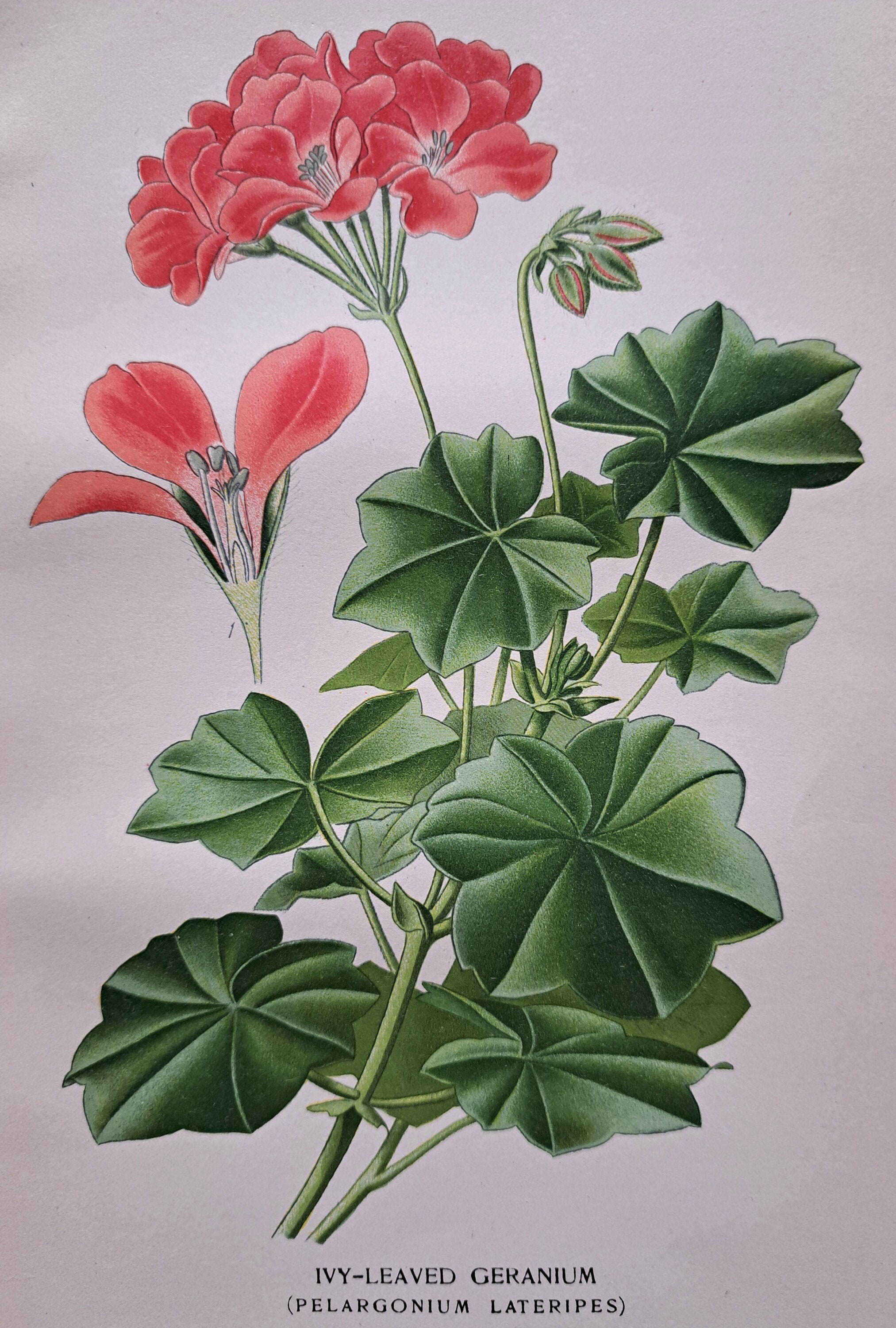The image is an educational-style, textbook-like illustration of a flower, likely a drawing or painting with a fairly realistic depiction. The background is primarily white, with a hint of a purple-pink hue blending in. The plant is an Ivy-leaved Geranium, or Pelargonium lateripes, as identified by the text at the bottom of the image. The flowers at the top of the stem are a striking dark pink with slight whitish edges, creating a tightly packed cluster. Some buds appear at the top, showing red tinges indicating they are yet to bloom. The green stem has large, rounded green leaves fanning out, each leaf featuring prominent, bold lines. A close-up cross-section of one of the flowers highlights its detailed interior, including the stamen.